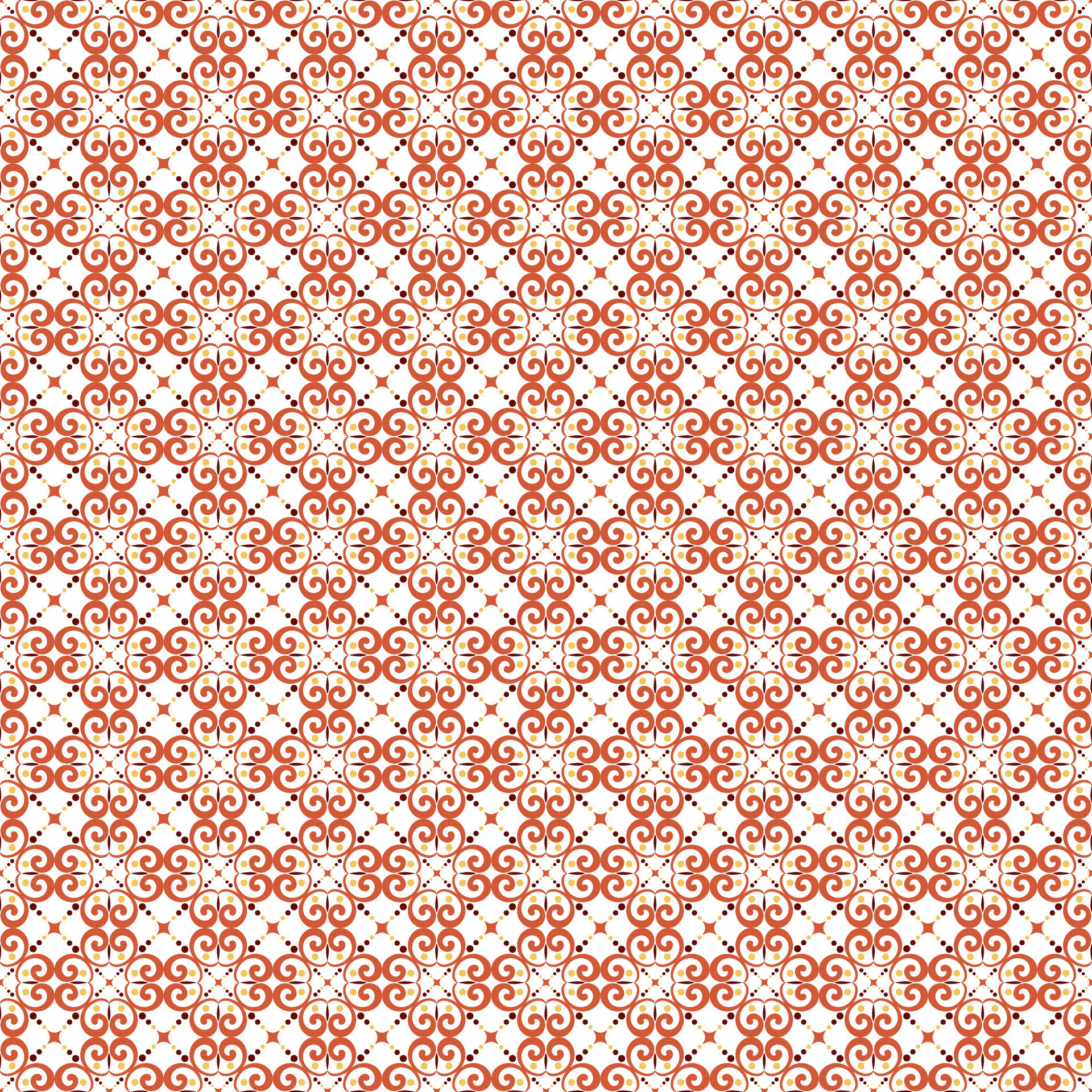This image showcases a complex, seamless, repeating pattern composed of grid-like units. Each unit features a central, four-pointed star in shades of orange and red, surrounded by symmetrical, intricate swirls. Dots, ranging from yellow to brown, radiate outward from the star, contributing to the overall intricate design. The swirls and dots create a lattice effect when viewed from a distance, forming a cohesive and elegant graphic pattern. The background is predominantly white, which enhances the visual contrast and detail of the red and orange swirling elements. This meticulous arrangement of repeated squares imbues the design with a sophisticated, almost gingham-like appearance.